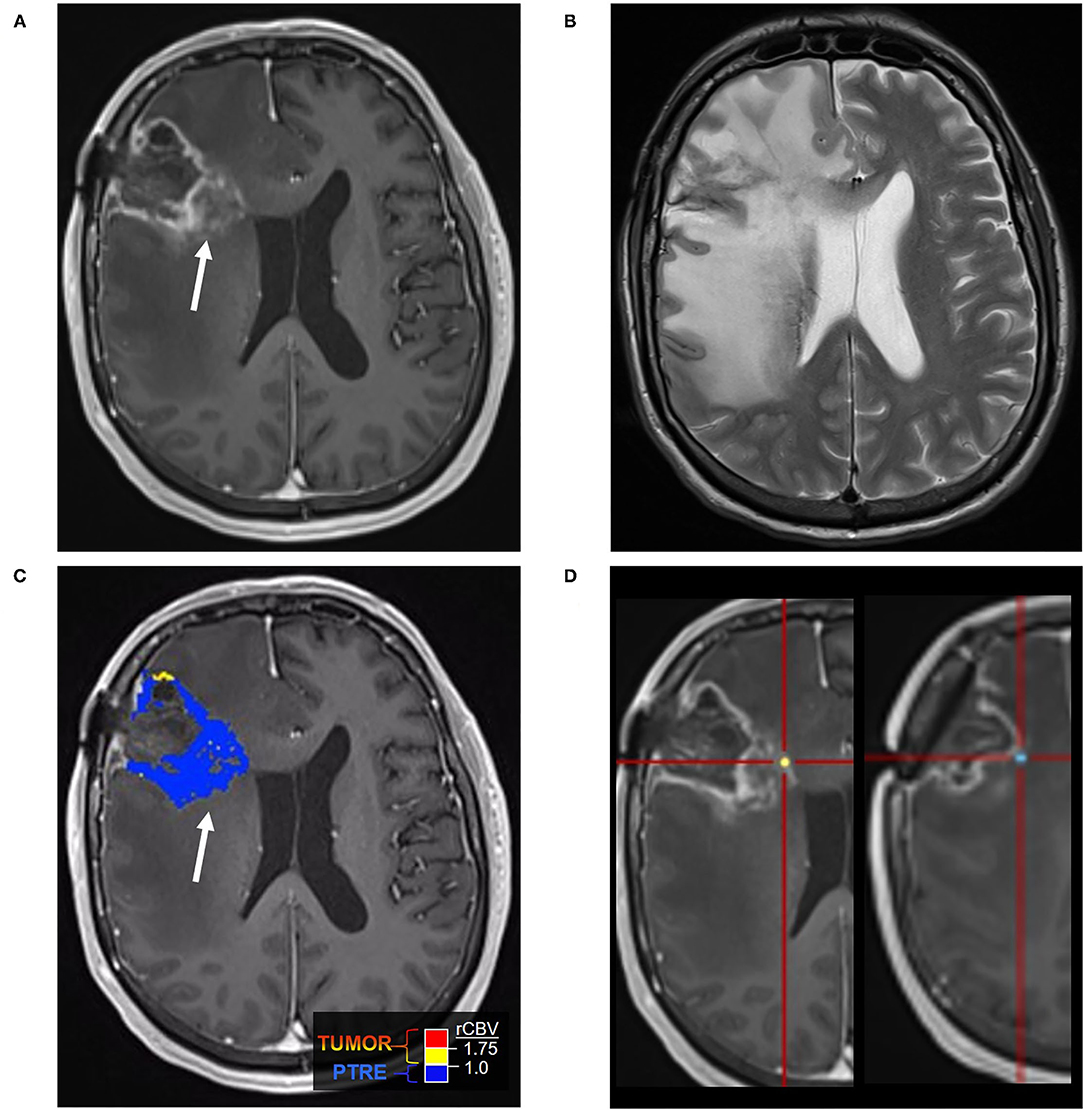The image depicts four horizontally arranged CAT scan images, each labeled A, B, C, and D, displaying detailed sections likely of a person's head or brain, all against a consistent black background. Image A, situated at the upper left, features a white border and a significant white arrow pointing to a specific section, implying an area of interest. To its right, Image B, distinguished by a black border, presents a white central area with lighter gray zones. The bottom left, Image C, also framed by a white border, prominently shows a blue-stained area indicated by an arrow, which is identified as a tumor, labeled 'P-T-R-E' with corresponding color blocks: red, yellow, and blue, as described in the legend. Finally, Image D on the bottom right appears to show split halves of the scan, marked with red crosses, suggesting targeted markers possibly for treatment considerations such as radiation. Overall, the images detail varying views and highlighted details within the scans, emphasizing the identified tumor and its precise locations through color-coded and marked annotations.